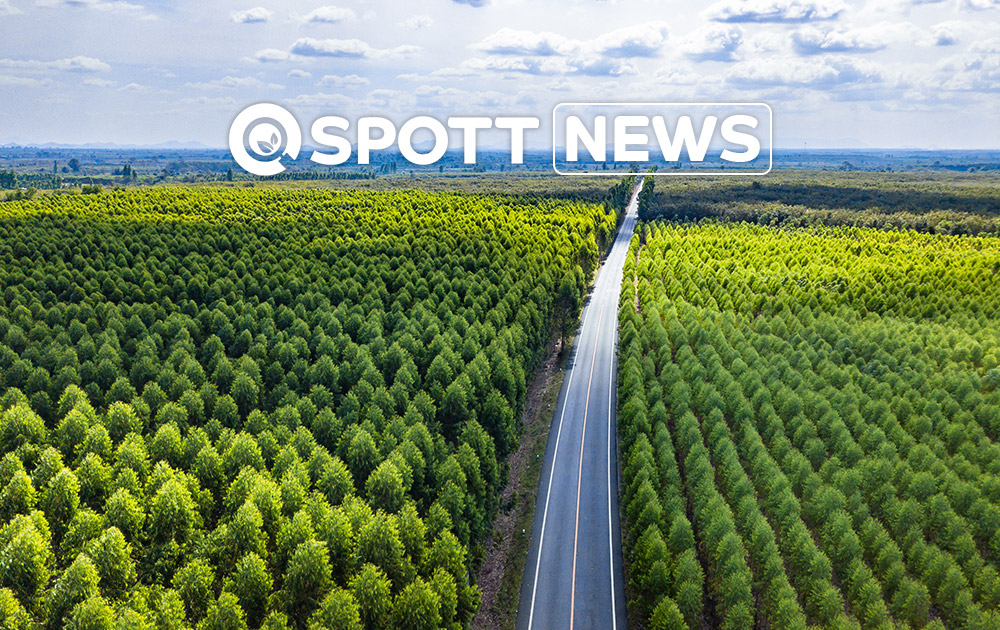This aerial photograph captures a sprawling landscape viewed from high above, with a prominently featured road cutting through the center. The road, paved and devoid of traffic, extends from the bottom center of the frame and disappears into the distant horizon, slightly curving as it recedes. It is marked by a solid yellow central line flanked by white edging lines, and the left shoulder appears wider than the right. On either side of the road, extensive rows of uniformly green, tapered trees stretch out endlessly, forming impeccably straight lines. Notably, a section on the right shows a distinct transition where the type of trees changes abruptly. 

The sky is crowded with various shades of gray clouds, casting soft shadows over the forested areas. Though the sky is predominantly overcast, there is a glimpse of blue on the horizon. In the top-center of the image, the words "Spot News" are prominently displayed in white, with "News" enclosed in a rectangular border. To the left of this text, there is a logo resembling a magnifying glass examining leaves, encircled by a white border. The minimalist, sky-dominated backdrop emphasizes the lush greenery and the solitary road, creating a striking balance between nature's expanse and human infrastructure.